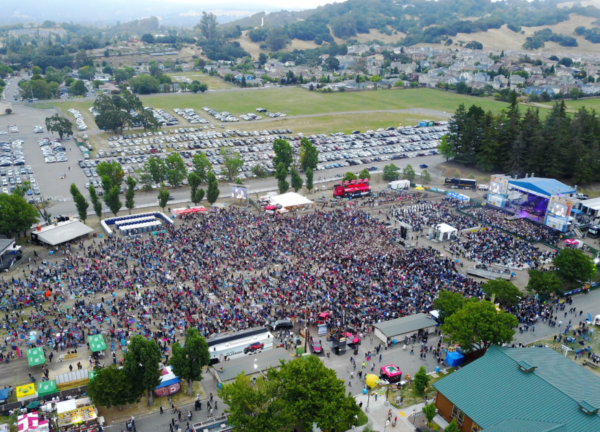This detailed aerial photograph, likely taken from a drone, captures the vibrant atmosphere of a daytime music festival set in a picturesque park surrounded by green rolling hills. The central element of the image is a massive crowd, possibly numbering around 5,000 people, gathered in front of a large stage situated on the right side of the frame. This stage, adorned with a blue roof and illuminated by purple lighting, anchors the event with the crowd stretching out across approximately a football field and a half.

Scattered throughout the festival grounds are smaller stages, food trucks, and vendor tents, selling gear and merchandise, creating a bustling perimeter. In the lower section of the image, a street lined with open shops and people walking contributes to the lively setting. Towards the top of the image, there are packed parking areas within fields and a designated parking lot, beyond which residential houses can be seen. The festival's location amidst these scenic hills emphasizes its expansive and communal nature. Additional trees and scattered attendees near the edges of the photograph enhance the overall festive and immersive experience captured in this expansive aerial view.